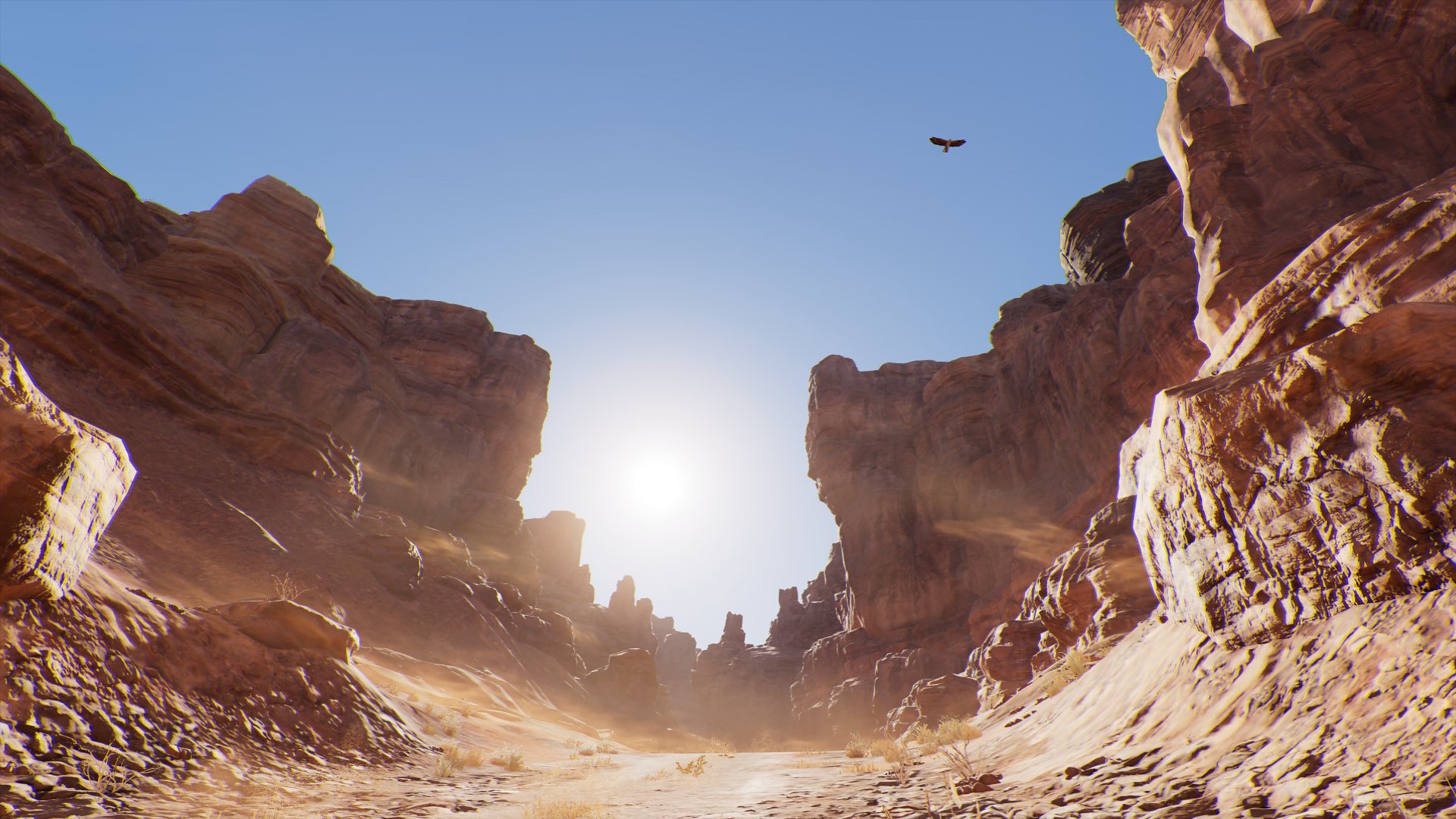This photograph, captured during the daytime, offers a breathtaking view down a dirt road nestled within a canyon. The perspective from the ground provides a unique vantage point of the brownish dirt path, flanked by rocky walls on either side. These rocks, imposing and rugged, extend into the background, gradually diminishing in size as they recede towards the horizon. Dominating the center of the sky is the radiant sun, which casts a reflective glow on the ground below, creating an ethereal and almost smoky effect. Adding a touch of life to this serene landscape, a bird—likely a hawk—soars gracefully in the upper right-hand corner of the sky.